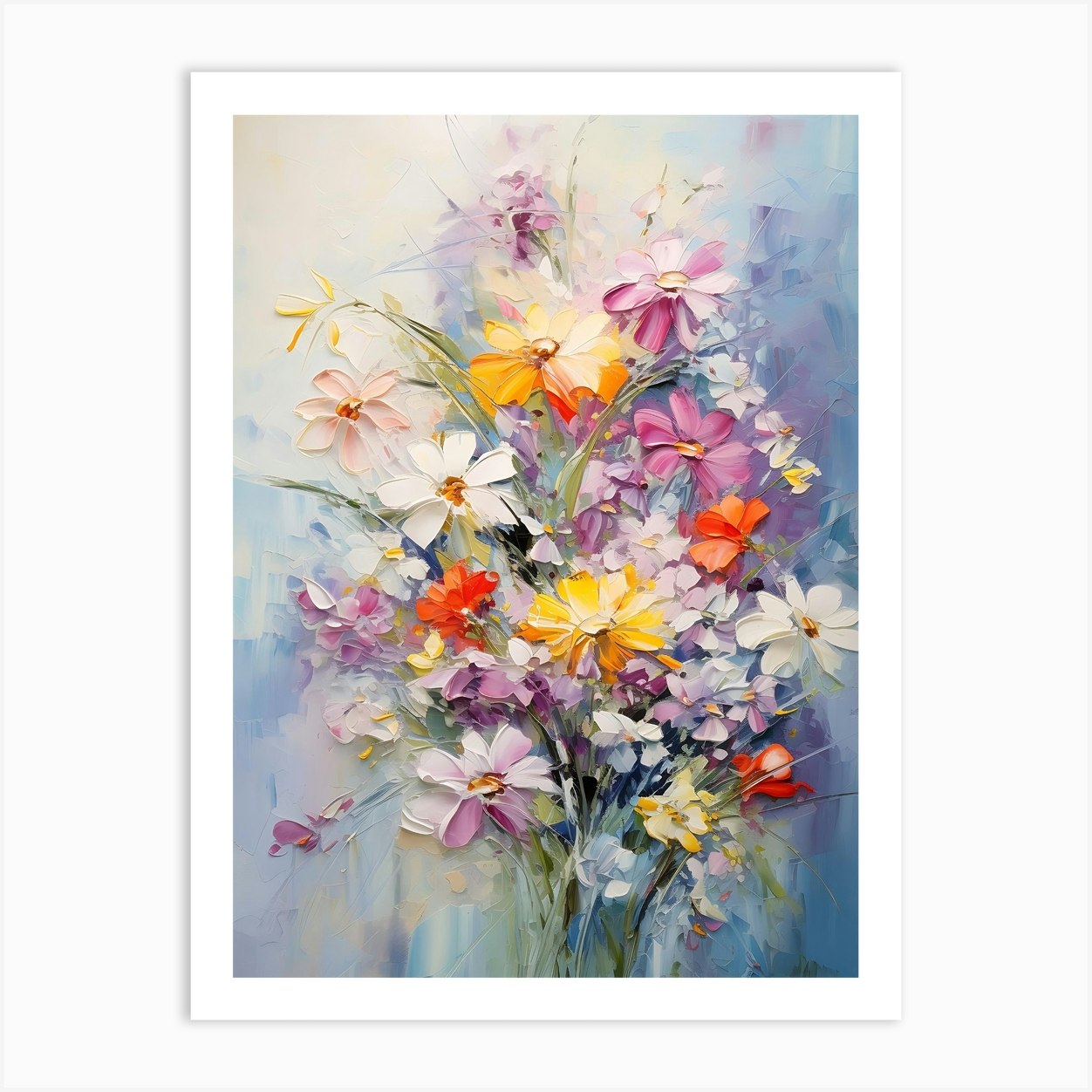This image features an exquisite painting, likely created with oil paint, depicting a vibrant bouquet of flowers. The flowers, reminiscent of daisies, are arranged in a crystal vase at the bottom of the image, from where they spread out elegantly. The background is a muted blend of white, blue, purple, and cream hues, becoming whiter on the left side and light blue on the right. The stems are a pale, light green and appear thin with minimal leaves. The bouquet includes flowers with yellow centers and white petals, yellow-orange petals, purple-pink petals, and a striking variety of blood orange to red and very light blue petals. Some flowers stand tall while others droop slightly, their different lengths creating a dynamic composition. The painting, adorned with a delicate white frame, captures the intricate beauty and vibrant diversity of the flowers, making it a captivating visual experience.